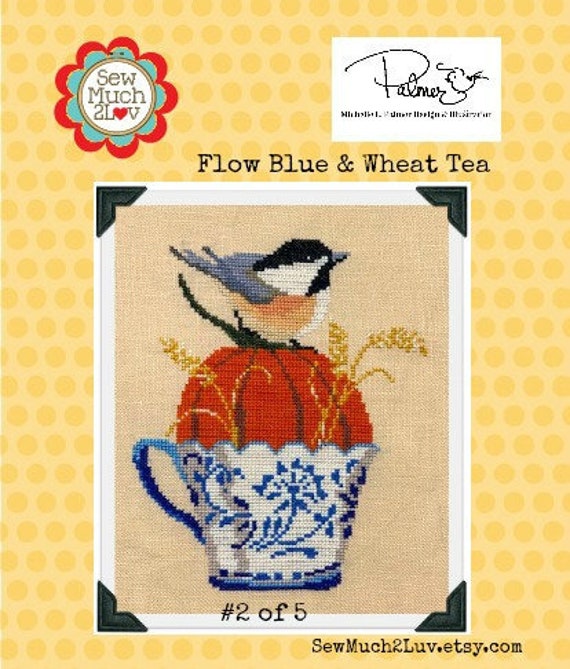This is an advertisement with a predominantly pale yellow background featuring a subtle honeycomb pattern made up of darker yellow dots. In the upper left-hand corner, there is a white circle outlined in yellow, surrounded by teal petals and then red petals at the tips. Inside the circle, it reads "so much to L" followed by a red heart and "V," completing the phrase "so much to love," with "sew" spelled as "S-E-W." To the right of this, in the upper right-hand corner, there is a white rectangle with the cursive signature "Palmer," ending with a small bird perched on the letter "R."

Below this, occupying the central portion of the image, is a framed cross-stitch pattern. The frame is white with black corners and is labeled "number two of five" at the bottom. Inside the frame, the pattern features a white teacup adorned with a blue floral chinoiserie design. Inside the teacup sits a dark orange pumpkin-shaped pin cushion with a green stem. Atop the pin cushion stands a bird with black, white, and orange feathers, resembling a chickadee. Above this framed design, in a serif-style typewriter font, it reads "flow blue and wheat tea."

At the very bottom right of the image, it says "so much to love.etsy.com."